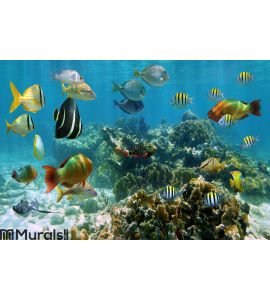The image depicts a vibrant underwater scene, which could be either a large aquarium or a shallow ocean area. The bottom of the image features a sandy and rocky seabed adorned with coral of various colors and sizes, including shades of green, orange, brown, and white. Prominently displayed in the lower bottom section is a striking fish with a green, yellow, and white body and a red tail. Above this fish, there is a thin, black-and-white striped fish. Towards the upper center, some fish resembling gray blowfish can be seen. To the right, an angelfish with distinctive stripes adds to the diversity. Several other colorful fish populate the scene, including medium-sized yellow-striped fish, larger gray fish with yellow tails, another large fish with two black stripes, and a vibrant rainbow-colored fish featuring orange, yellow, green, and black hues. The background water is a clear, medium blue, lending a crisp backdrop to the myriad of aquatic life. In the bottom left corner, the word "murals" is printed in black, alongside a indistinguishable logo, enhancing the artistic feel of the image. Light filtering into the water adds a natural luminance, suggesting the possibility of outdoor light, whether the scene is within an aquarium or in the wild.